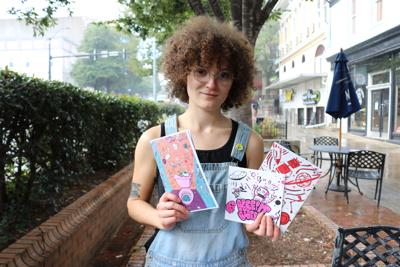The image features a young woman with very curly, afro-like hair and a fair complexion. She is wearing round-framed glasses and has a small tattoo on her upper left arm. She is dressed in light blue denim overalls over a black tank top. In her hands, she holds three colorful cards or flyers; one depicts a toilet, another a robot with the phrase "Keep it weird," and the third has a black and white design. The cards are vibrant, with prominent pinks, reds, blues, and purples, suggesting artistic or cartoon-like illustrations. She stands on a shiny, wet brick pathway, suggesting recent rain, near a row of bushes planted in a concrete planter. To her right are metal tables and chairs for outdoor seating, and behind her, there are storefronts, indicating she is in a retail or café area. A tree stands immediately behind her, adding to the scenic setting.